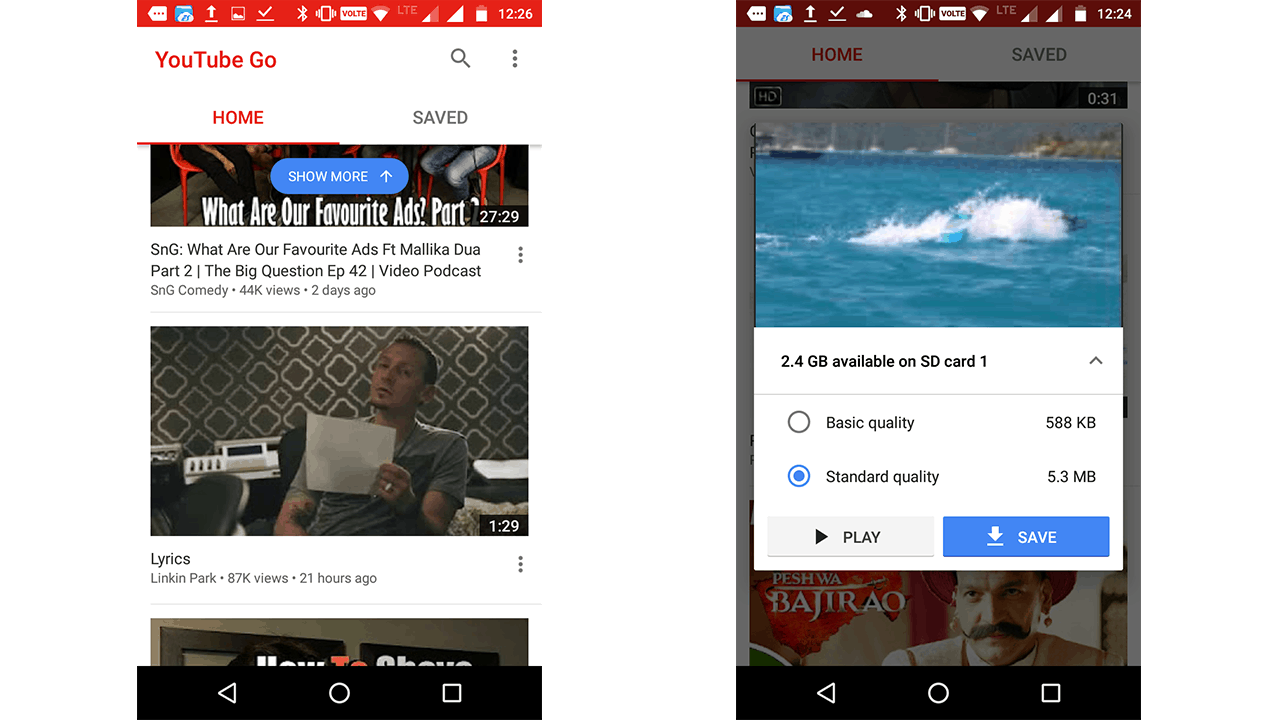The images show two screenshots of the YouTube Go app, an older version of YouTube. The notification status bar at the top of the screen is red, featuring an array of icons, including a picture icon, upload icon, Bluetooth icon, vibration mode icon, battery icon, and a clock showing the time as 12:26 PM on the right side.

Below the status bar, the main interface of the app has a white background with the "YouTube Go" logo prominently displayed in red on the left. Below the logo are two tabs: "Home," which is highlighted in red, and "Saved," which is grayed out. 

In the first screenshot, two videos are visible. The first video is titled "What are your favorite ads? - Featuring Malika Dua" by SNG Comedy, posted two days ago, with 44 views and a duration of 27 minutes and 29 seconds. The second video is a music video from Linkin Park with 87,000 views, posted 21 hours ago, and lasting 1 minute and 29 seconds. The thumbnail for the second video features the band’s lead singer.

The second screenshot, also from the YouTube Go app, similarly showcases the app's interface but highlights a different video. A pop-up box is prominently displayed, divided into two sections. The top section of the pop-up features an image of a splashing body of water, colored in aquamarine, reminiscent of a swimming pool or lake. Below the image, text indicates, "2.4 gigabytes available on SD card 1." Two download quality options are provided: "Basic Quality" for 588 KB, and "Standard Quality" for 5.3 MB, with the latter selected, marked by a blue bubble. At the bottom of the pop-up are two buttons: a "Play" button and a "Save" button, the latter button highlighted in blue.